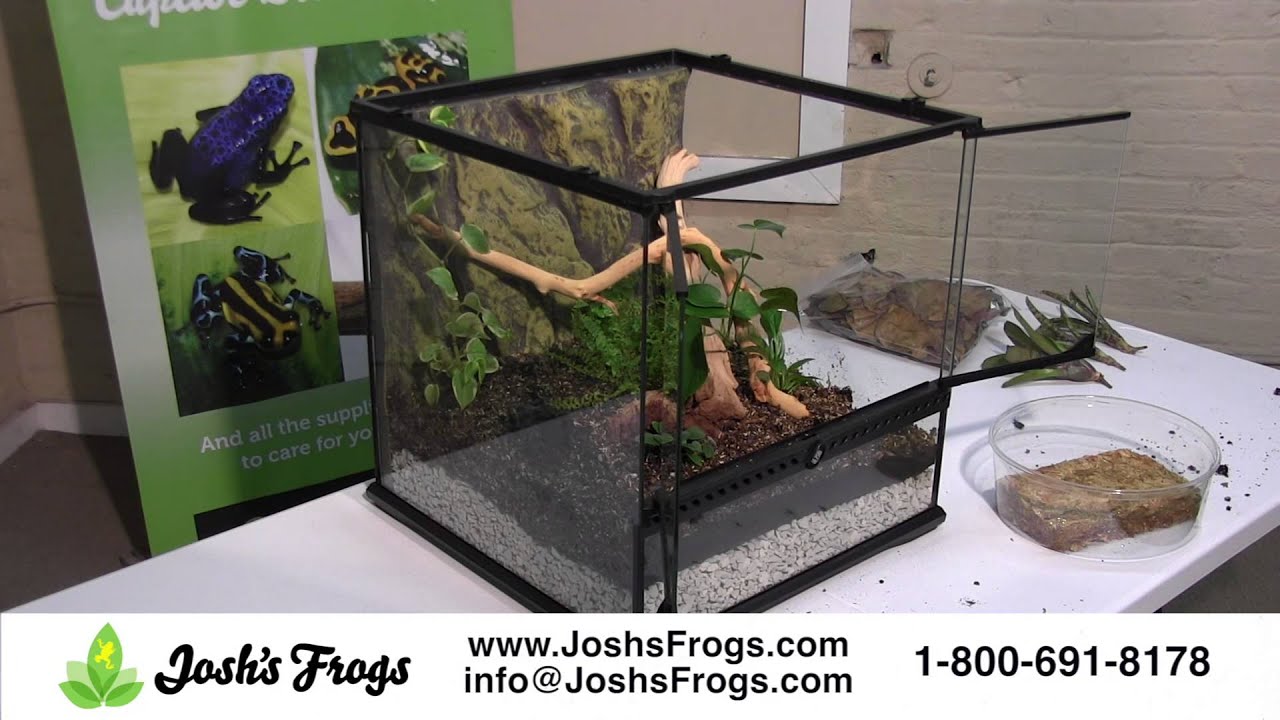The image showcases an advertisement for Josh's Frogs, a pet store specializing in reptiles. The focal point is a square acrylic terrarium placed on a white table, designed to resemble a tropical habitat with features such as green plants, a fern, and realistic tree branches. The bottom layer of the terrarium contains a gray, gravelly material topped with brown soil mixed with white perlite. Inside the tank, there's a medium-sized frog.

Behind the terrarium is a large green banner with multiple images of frogs displaying various color patterns, including blue, yellow, and black. The banner prominently advertises Josh's Frogs. At the bottom of the image, a white strip contains key contact information: the store's name "Josh's Frogs," the website "www.joshsfrogs.com," the email "info@joshsfrogs.com," and the phone number "1-800-691-8178." Additionally, there is an emblem featuring a five-leaf motif with a frog in the center.